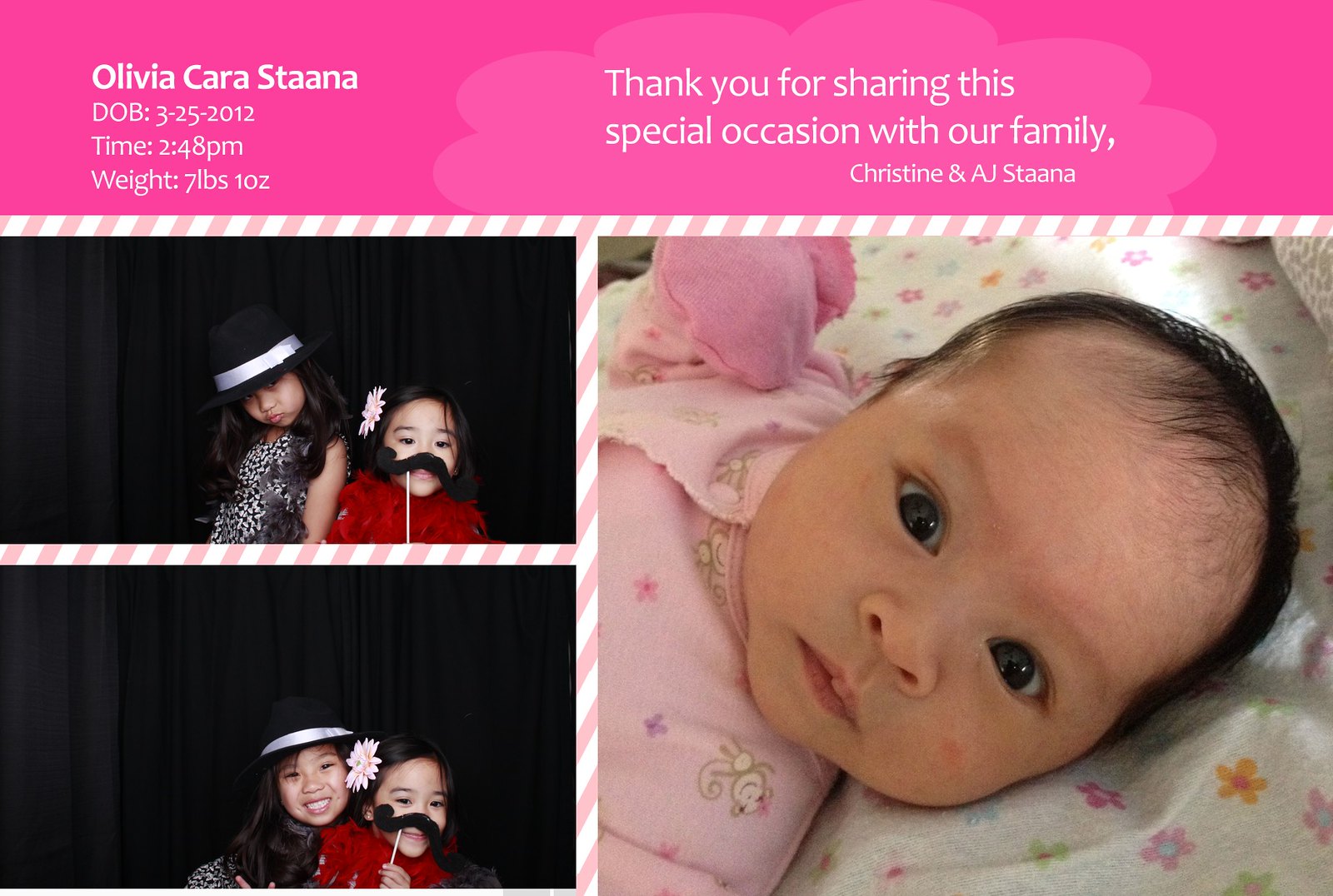The birth announcement is a rectangular thank-you card featuring three photographs, celebrating the arrival of Olivia Karastana. At the top of the card, enclosed within a pink border and white cloud-like background, the text reads: "Thank you for sharing this special occasion with our family, Christine and AJ Stana." Below this, Olivia's birth details are provided in pink text: "Olivia Karastana, DOB 3/25/2012, Time: 2:48 PM, Weight: 7 pounds 10 ounces."

The right side of the card prominently displays a large picture of a baby girl, Olivia, dressed in pink and lying on a flowered blanket. Olivia has dark hair. On the left side, two older girls are pictured. One girl is wearing a top hat and a black and white dress, while the other sports a pretend mustache, a flower in her hair, and a red boa. Together, these elements form a heartwarming and detailed introduction to the newest member of the Karastana family.